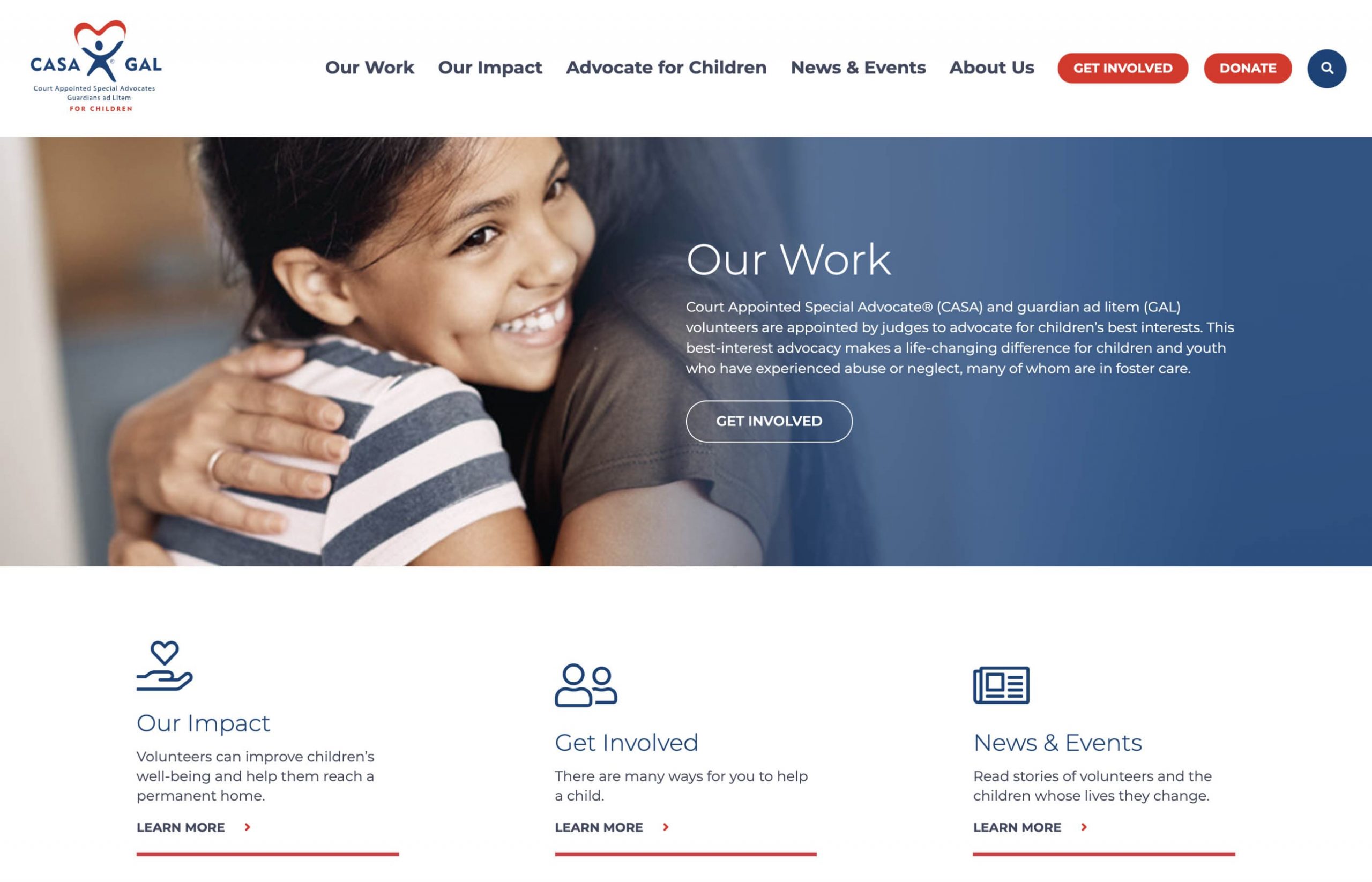Screenshot of CASA-GAL Website Overview:

The image captures a screenshot of the CASA-GAL website, showcasing the organization's dedication to advocating for children. At the center of the page, there's a touching photo of a woman warmly embracing a smiling young child, accompanied by the text: "Our Work, Court Appointed Special Advocate (CASA), and Guardian ad Litem (GAL). Volunteers are appointed by judges to advocate for children's best interests. This best interest advocacy makes a life-changing difference for children and youth who have experienced abuse or neglect, many of whom are in foster care."

Below this central message, there's a prominent "Get Involved" button inviting users to take action. Further down, three clickable options, "Our Impact," "Get Involved," and "News and Events," each have a "Learn More" prompt for additional information.

The top navigation bar provides links to sections titled "Our Work," "Our Impact," "Advocate for Children," "News and Events," and "About Us." On the far left side of the page, there are additional buttons labeled "Get Involved," "Donate," and a search option for easy website navigation.